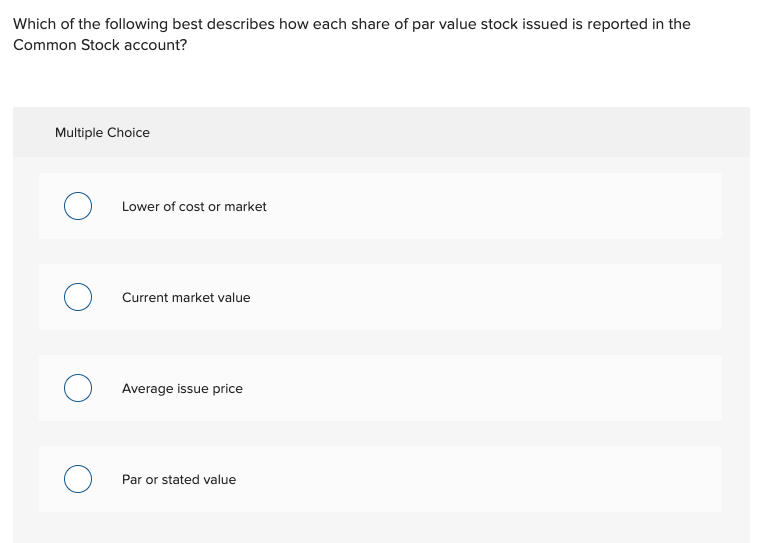The image features a query regarding the financial reporting of PAR value stock. The top section of the image has a white background with the text "WHICH OF THE FOLLOWING BEST DESCRIBES HOW EACH SHARE OF PAR VALUE STOCK ISSUED IS REPORTED?" written in black, bold capital letters. Below this, the text "COMMON STOCK ACCOUNT?" appears in black, with only the first letters capitalized.

Below this question, there is a gray rectangle. On the top-left corner of this rectangle, the words "MULTIPLE CHOICE" are displayed in black, with each letter in "MULTIPLE" and "CHOICE" capitalized.

Inside the gray rectangle, there are four blue-outlined, white circles that resemble radio buttons used in online forms or tests. These circles can typically be selected to indicate a choice, potentially turning black or blue when selected. Each circle is accompanied by an answer option written in black text:

1. "Lower of Cost or Market" with the first letters capitalized.
2. "Current Market Value" with the first letters capitalized.
3. "Average Issue Price" with the first letters capitalized.
4. "PAR or Stated Value" with the first letters capitalized.

Although there are options to be selected, there is no visible mouse pointer in the image to indicate a current selection.

This setup illustrates a typical format for a multiple-choice question related to accounting, specifically focusing on the reporting of issued shares of PAR value stock.